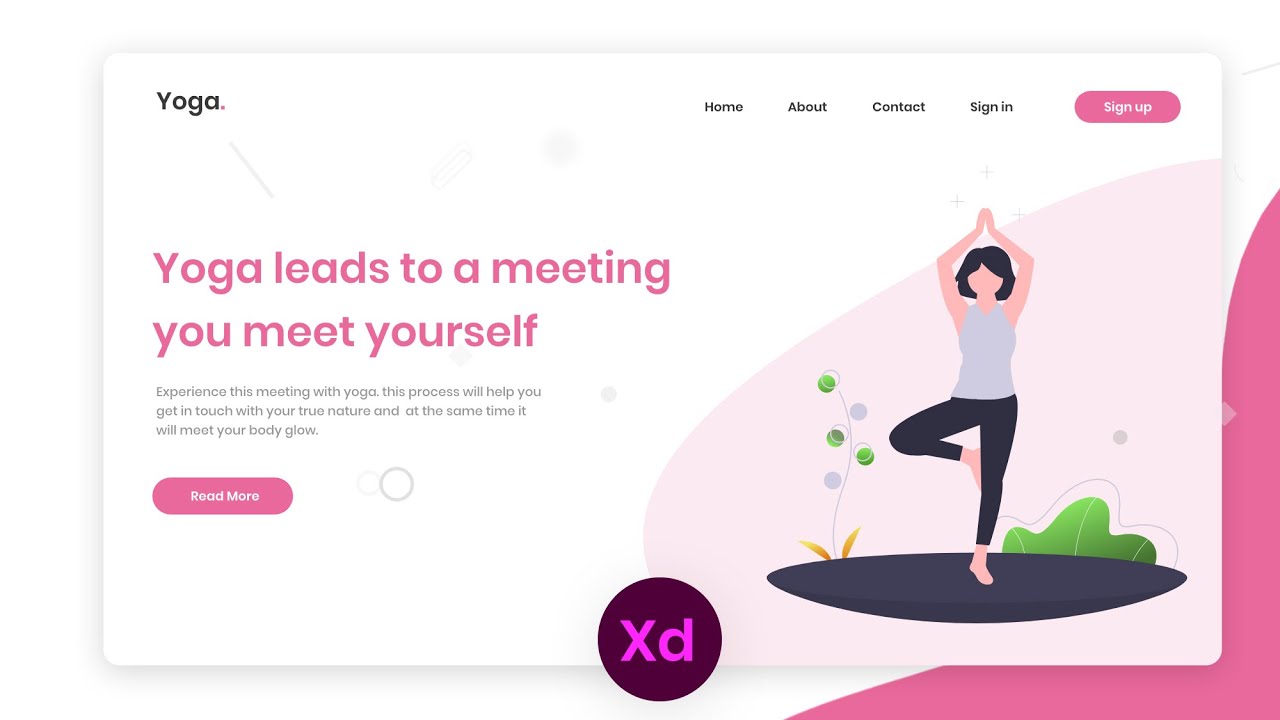The screenshot features a predominantly white background with a large white rectangle prominently displayed. In the upper left-hand corner, the word "Yoga" is written in bold black font. Centered near the top, there is a horizontal navigation menu with the items "Home," "About," "Contact," and "Sign In." Adjacent to the menu is a pink oval button with white text that reads "Sign Up."

Midway down on the left side, in large pink letters, the text reads, "Yoga leads to a meeting. You meet yourself." Below this, in black text, it says, "Experience this meeting with yoga. This process will help you get in touch with your true nature and at the same time, it will make your body glow." Approximately three lines below this text, there is another pink oval button with white text that says "Read More."

Positioned towards the lower half of the image, there is a faint pink patch that curves upwards and to the right. A computer-generated image of a woman is situated here, characterized by short dark hair and raised arms with palms meeting above her head. She is in a yoga pose, balancing on her left leg with her right foot pressed against the inside of her left knee, standing on a black circle. A hot pink patch accents the image, flowing from the lower left-hand corner and extending up along the right edge.